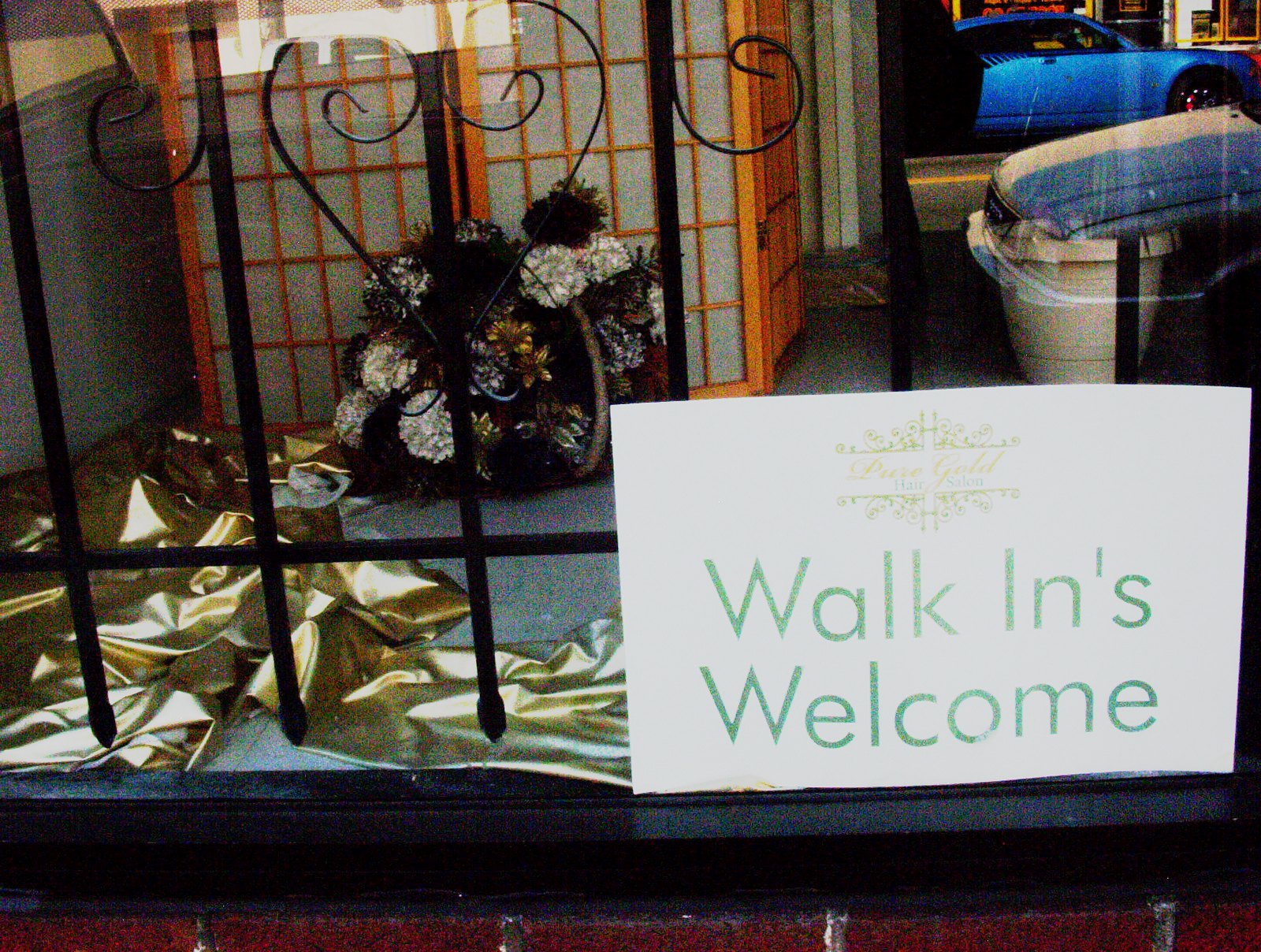This photograph captures the elaborate exterior of a shop, identified as Pure Gold Hair Salon, through a glass window adorned with an ornate black metal fence. In the bottom right corner of the window, a white sign reads "Walk-ins Welcome" in green font below the salon's gold logo, "Pure Gold Hair Salon." Inside the window, a luxurious display includes a gold tarp or ribbon on the ground, festive gold and white bows, and a brown lattice structure with windows at the center-left, complemented by a vibrant array of flowers in front. Reflections in the glass faintly capture city street elements, including parked cars, enhancing the image's bustling, urban ambiance.